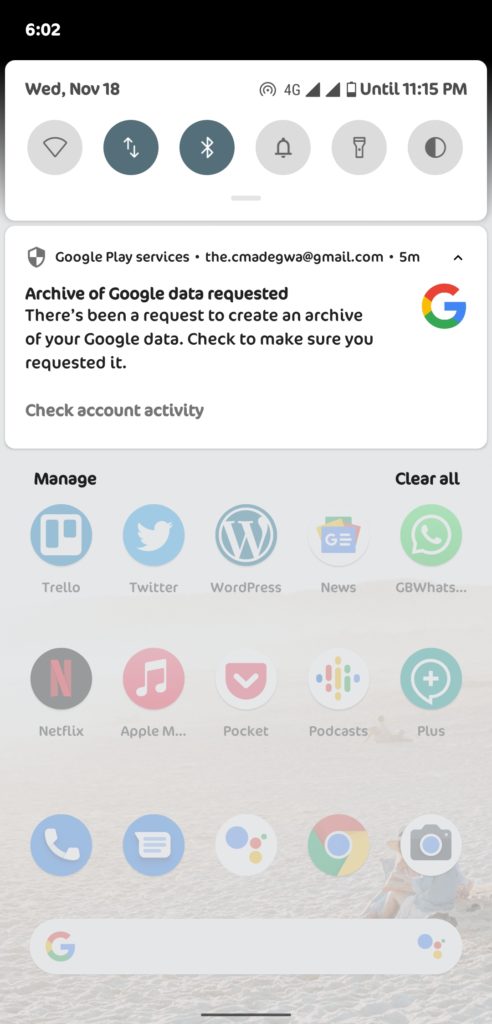Screenshot of an Android Cell Phone Screen

The image is a detailed screenshot taken from an Android cell phone display, showcasing the interface with precise clarity. The time is prominently displayed as 6:02. Below the time, a control box features various user options in a vertical arrangement. 

Highlighted controls include:
- **Wi-Fi**: Represented by a gray circle, indicating it's off. The Wi-Fi icon shows an empty triangle with a curved bottom, devoid of signal strength bars.
- **Mobile Data**: Depicted by a dark bluish-green circular icon with upward and downward arrows nearly touching at the center, indicating it is activated.
- **Bluetooth**: An activated icon illustrated with the standard Bluetooth symbol.
- **Notifications**: A gray bell icon, signifying no notifications.
- **Flashlight**: Another gray icon illustrating a flashlight.
- **Contrast Setting**: A gray icon split into half black and half white or unfilled, likely indicating a contrast setting.

In the top left corner, the date and time details are given as "WED, NOV 18" in red. Adjacent to this are various status icons, including:
- **4G**: Alongside two full signal strength icons and a battery icon showing about 25% charge, with a note stating "until 11:15 PM."

The following section displays a notification from Google Play Services linked to the email d.cmadegwa@gmail.com received five minutes ago. The notification reads:
- **Bold Text**: "Archive of Google Data Requested."
- **Standard Text**: "There's been a request to create an archive of your Google data. Check to make sure you requested it."
- **Gray Text**: "Check account activity."

To the right of this notification is the multi-colored Google "G" logo, followed by "Manage" and "Clear All" in bold black text, appearing on the left and right sides respectively.

Below the notification, several app icons are visible, albeit slightly obscured by a gray foggy texture:
- **Trello, Twitter, WordPress, Google News, WhatsApp (gbwhats...), Netflix, Apple Music, Pocket, Google Podcasts**.
- The following apps are without text labels: **Phone, Messaging, Google Assistant, Google Chrome, and Camera**.

At the bottom, the Google search bar is present. The background image of the phone, partly obscured by the camera icon, seems to depict a beach scene.

This comprehensive screenshot captures the functional and aesthetic elements of the Android interface, neatly organizing various controls, notifications, and app icons over a subtle beach-themed wallpaper background.